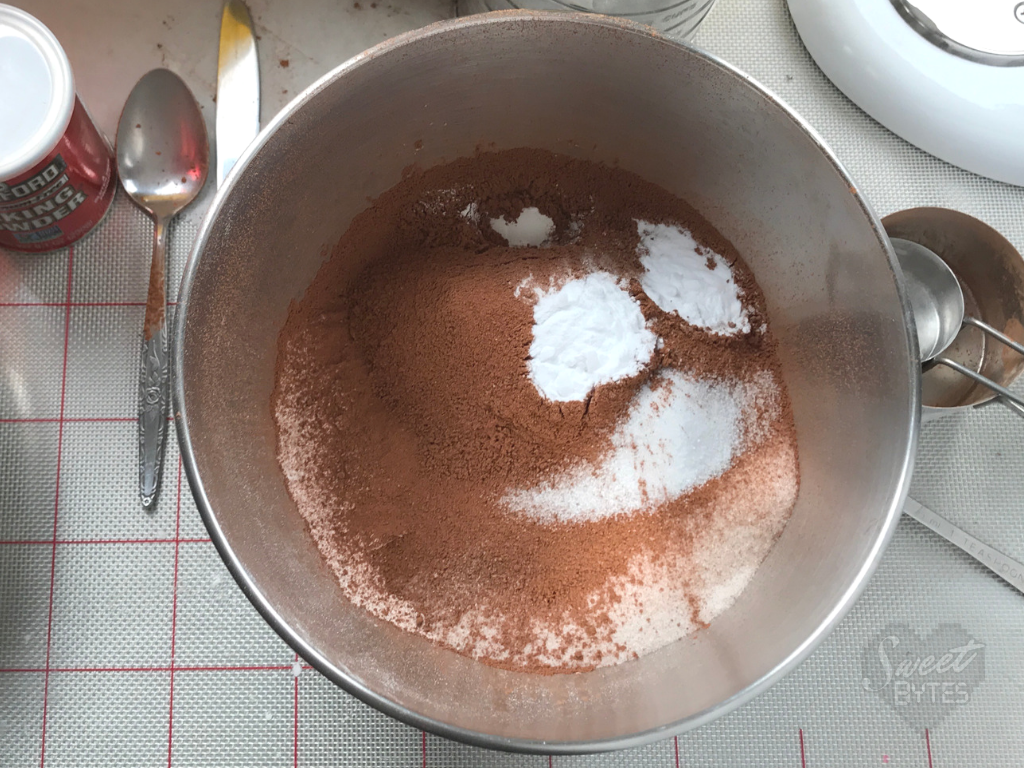The image is a top-down view of a chrome-colored metal mixing bowl resting on a kitchen surface, filled with dry baking ingredients. Inside the bowl, there are distinct portions of brown powder, likely cocoa powder, and white powder that could be sugar, baking powder, or flour. Some of the ingredients are mixed, revealing a blend of brown and white powders. A metal spoon with a flowery design on the handle, bearing traces of brown powder on the stem, lies to the left of the bowl. To the right, a set of measuring cups containing similar brown and white powders can be seen. In the top left corner, there is a small red can with a plastic lid, which seems to be labeled "baking powder." Below the bowl, there is a text or label that reads "sweet bites," with "bites" spelled "b-y-t-e-s," hinting at a playful theme related to baking. The overall setup suggests preparations for baking, possibly a chocolate cake, evidenced by the presence of cocoa powder and other typical baking ingredients.